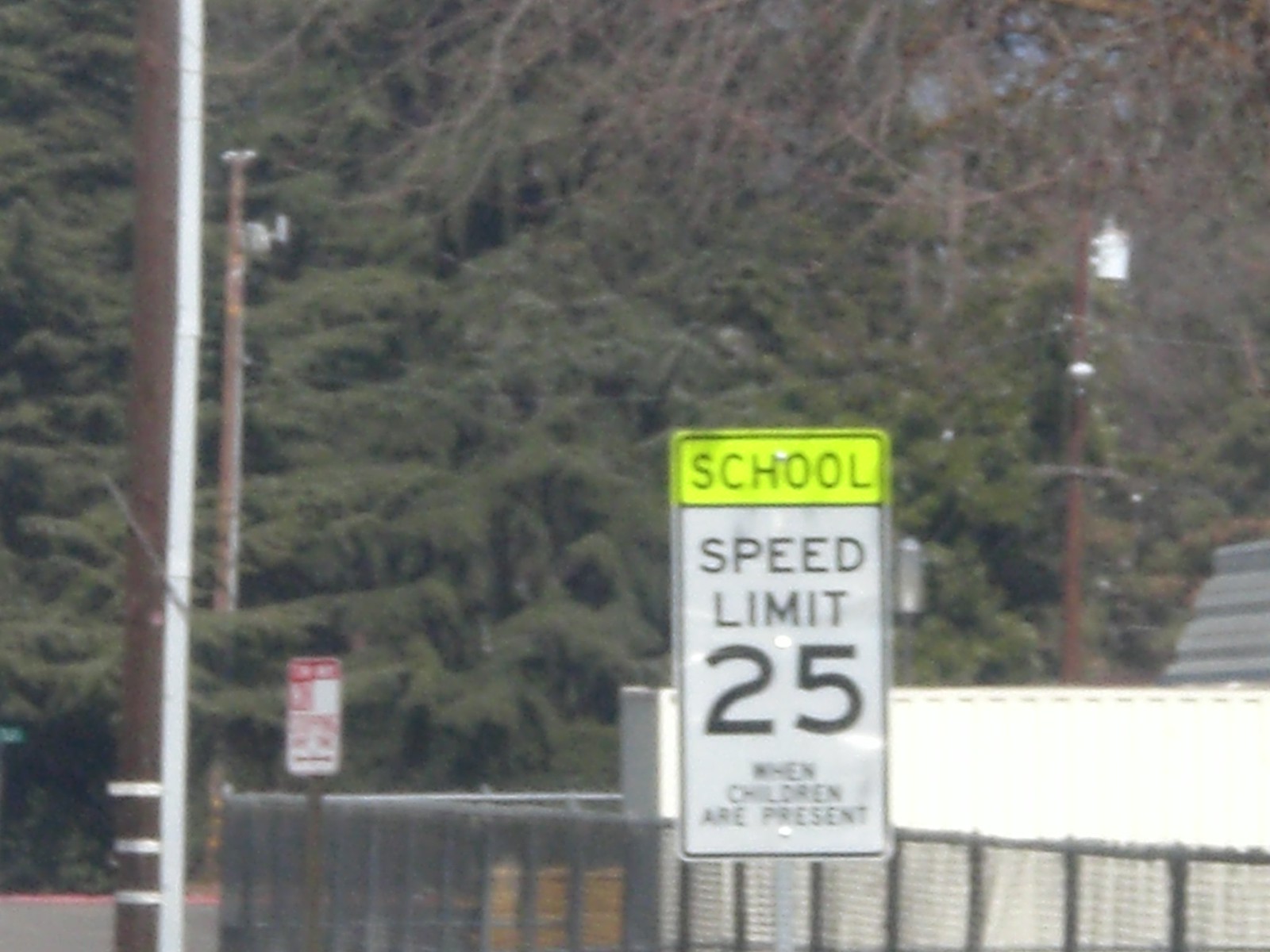The photograph depicts a rectangular school zone sign mounted on a silver post. The top section of the sign features the word "SCHOOL" in black font against a neon yellow background. Below that, another sign dictates "SPEED LIMIT 25" in black font on a white background, followed by the words "WHEN CHILDREN ARE PRESENT." 

Adjacent to the sign, on the left side of the frame, a telephone pole extends from the bottom up to the edge of the photograph, intersected by another telephone pole in the background. Numerous pine trees populate the backdrop, along with a barren tree situated in the upper right corner and another telephone pole near it. 

A gray roof is partially visible toward the middle right side of the image. At the bottom of the frame, a silver chain-link fence runs horizontally behind the school zone sign. Additionally, a red and white rectangular sign can be seen in the distance.